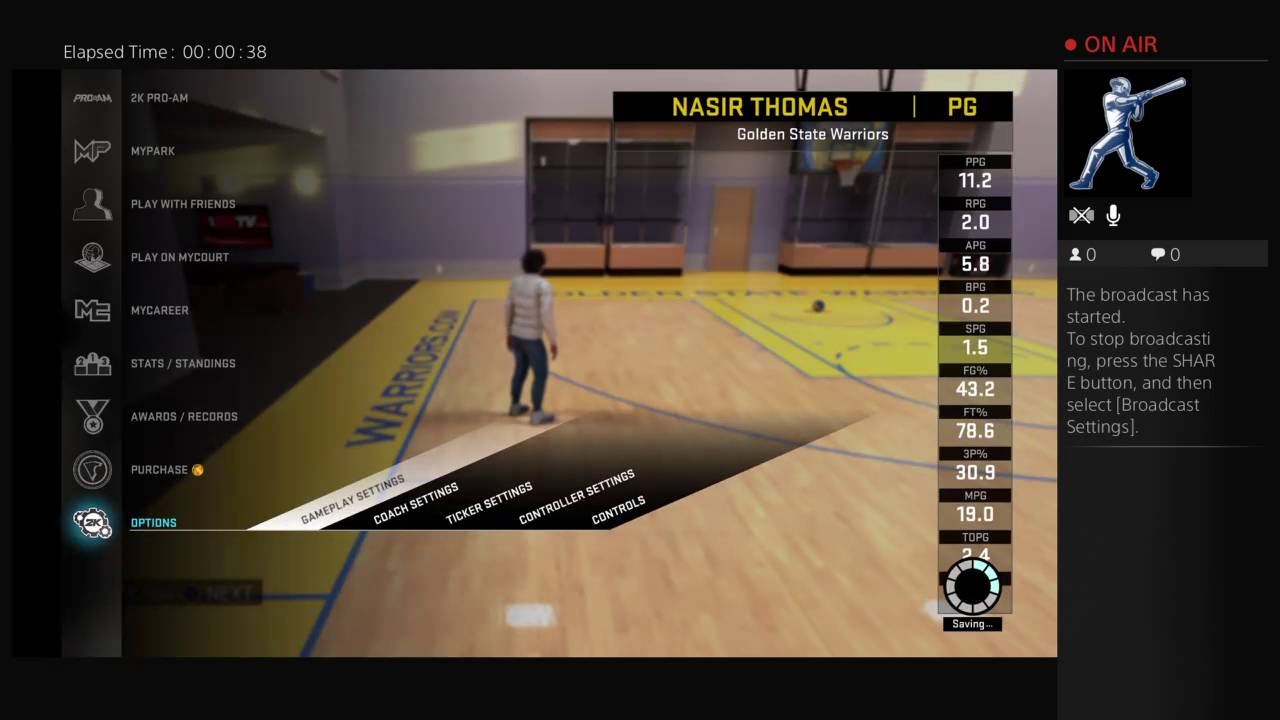The image is a screen capture from an online game simulation featuring a detailed 3D-rendered scene. Dominating the black background is a large visible image frame showcasing a person in black pants and a cream-colored top, standing on a basketball court. The court's hardwood floor is light brown, accented with yellow boundary lines. Along the vertical side of the yellow border, the word "Warriors" is prominently written in blue. In addition to the main scene, the screen includes white text and numbers dispersed across it. To the right side, beneath a black bar displaying the name "Thomas Nasser" and the position "PG," a column of various score points is listed in white. This comprehensive layout provides a realistic and immersive gaming experience.